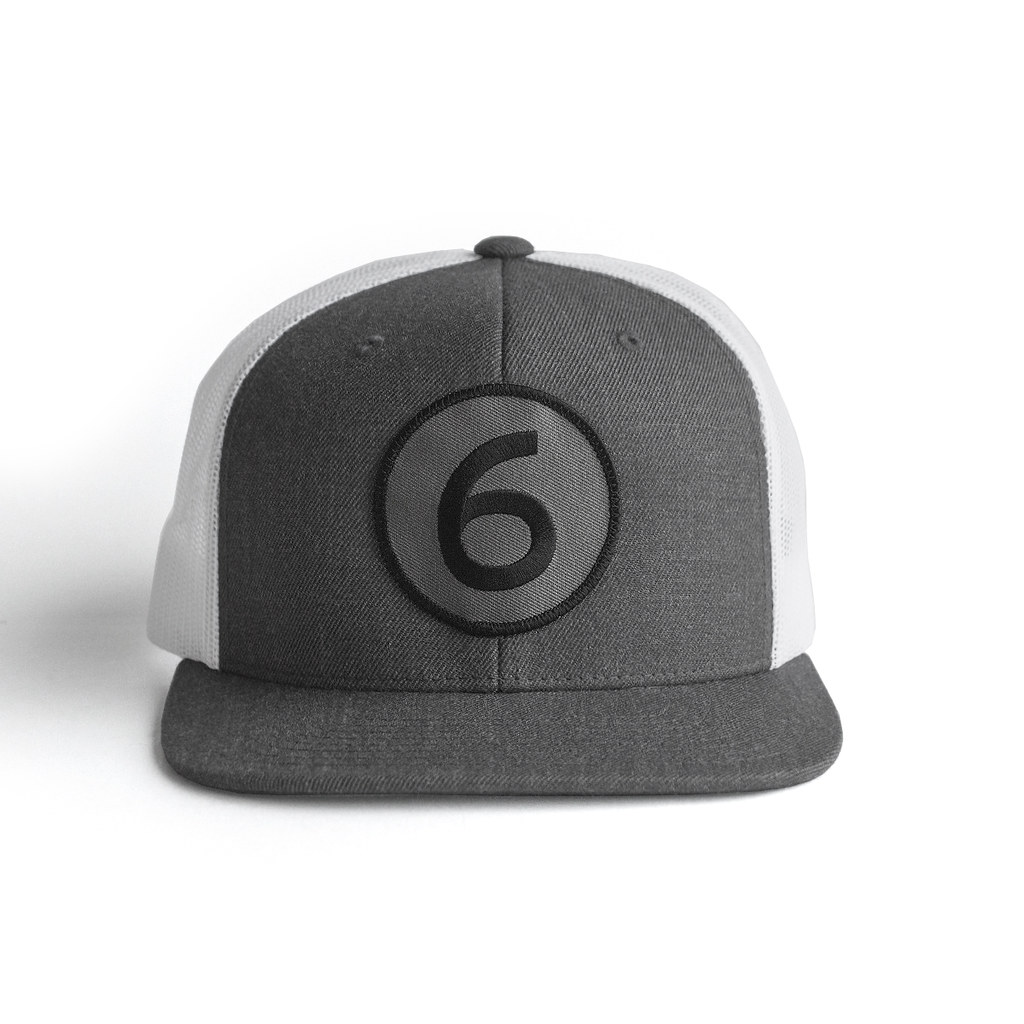This high-quality studio photograph features a baseball-style cap, prominently showcasing its detailed design against a pristine white background and surface. The cap is positioned with its dark gray brim facing forward, resting flat. The front of the cap, also dark gray, is centrally divided by a seam that runs from the top to the brim. At the apex of this seam is a matching dark gray button. The center front panel features a distinctive black circle with a thick black number "6" inside, set against a slightly lighter gray background. The sides of the cap are white, accentuated by the seams that neatly separate the different colored panels. Although the back of the cap is not fully visible, it appears to be made of a white mesh material. A faint shadow is cast towards the back left corner of the image, adding a subtle depth to the composition.